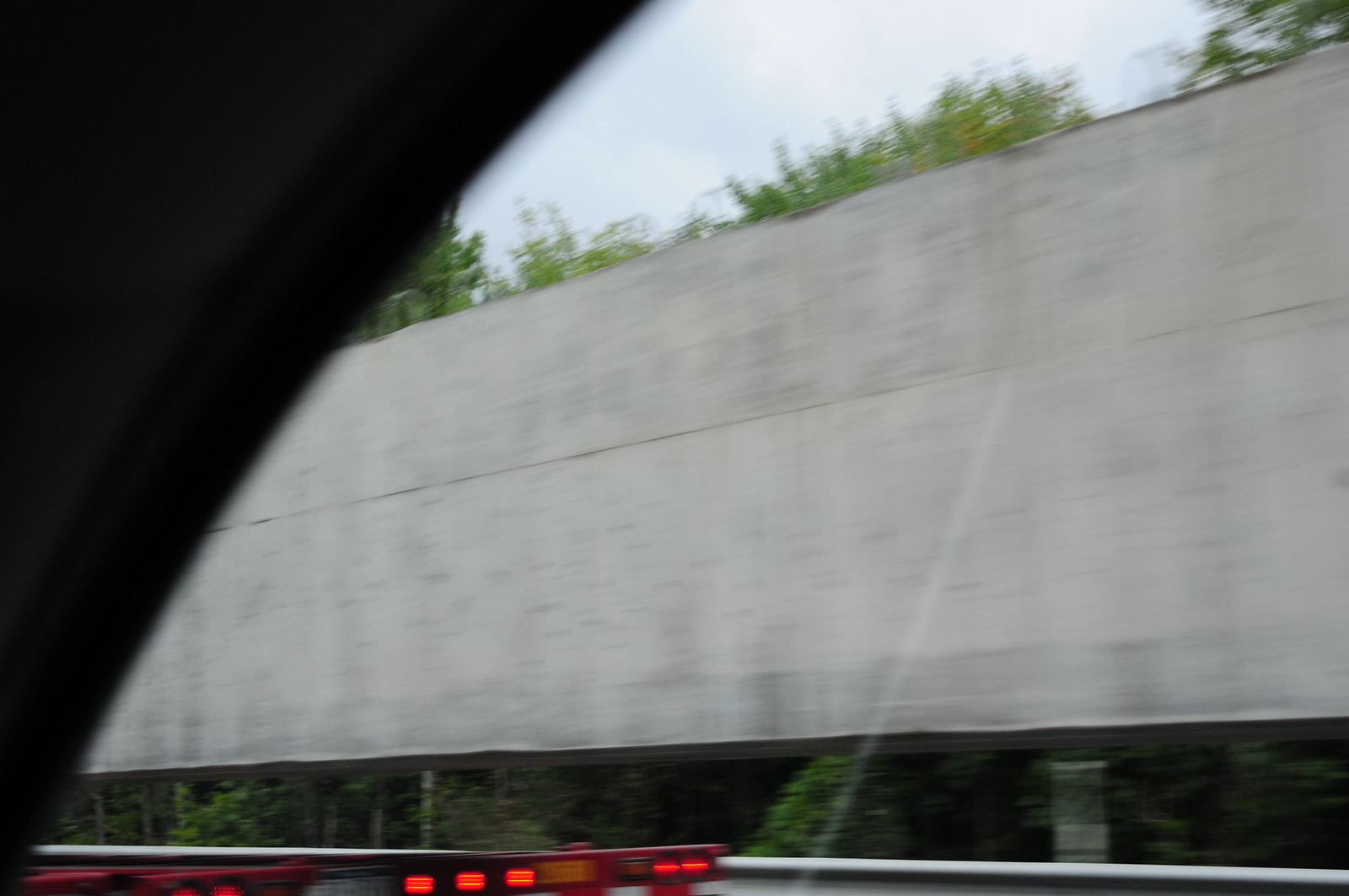A view from the passenger seat of a vehicle captures the scenery through the window. The upper left corner features a dark gray, curved contour where the window meets the windshield. Outside, a flat gray wall extends across the middle of the image, topped and bordered by verdant green foliage. Beyond this wall, more greenery is visible. The sky above is a mix of light blue and white cloud cover. In the foreground, the lower left section reveals the red back end of a flatbed truck, prominently displaying five glowing red brake lights.